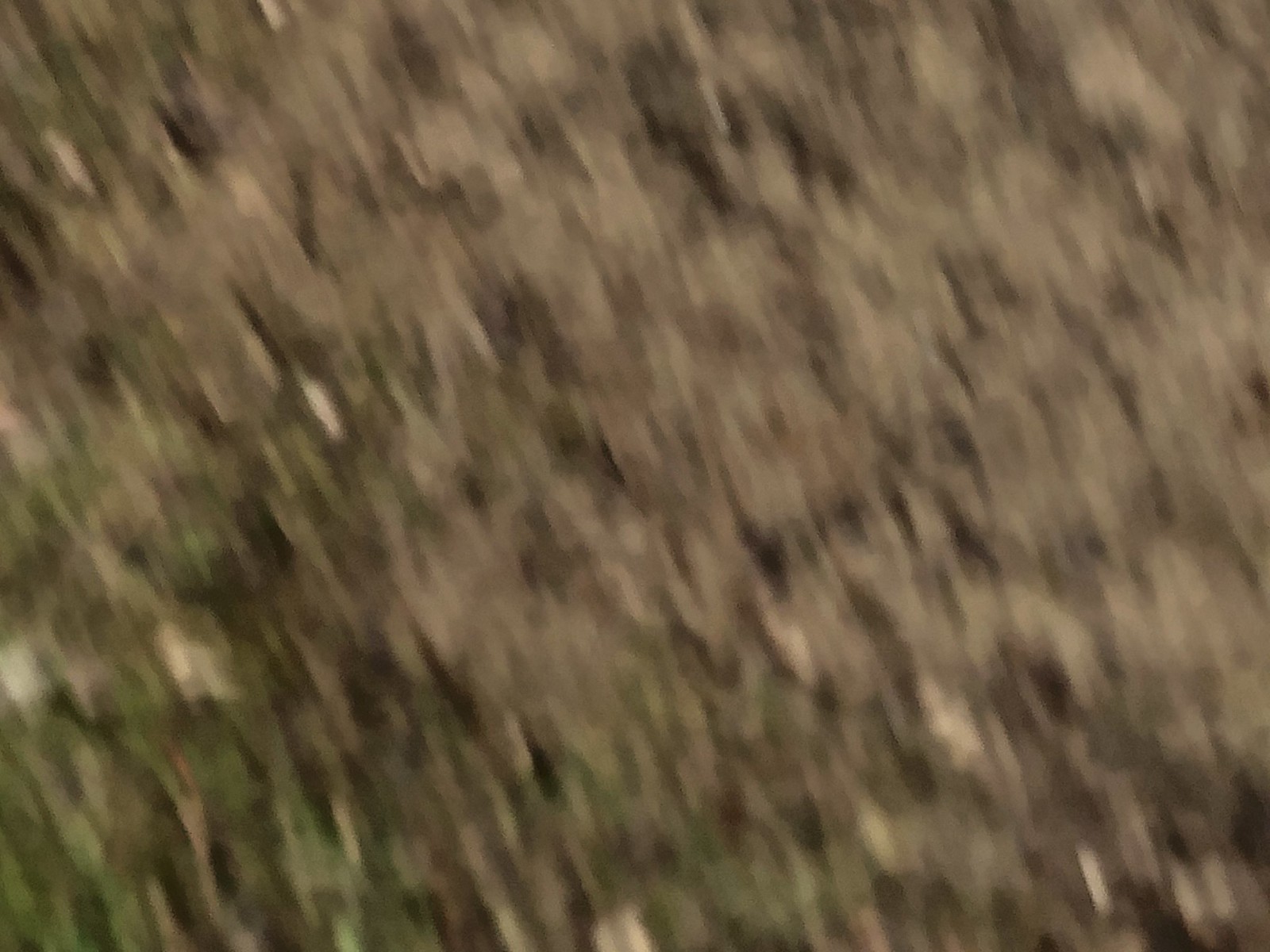This is an abstract, blurry photograph of the ground, likely taken accidentally. The image captures a mix of green grass interspersed with brown earth, suggesting either a parking lot or a forest path as the setting. The left side of the photograph features more greenery, with patches of moss and grass, though overall, the scene appears somewhat dirty and unkempt. The photograph, appearing grainy, suggests it was taken in well-lit, daytime conditions. Despite the lack of sharpness, some indistinct elements like rocks and leaves are faintly visible on the ground.